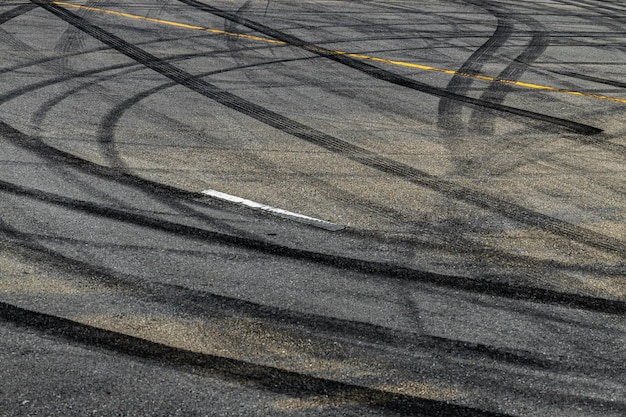The image depicts a heavily patterned pavement, likely a section of a street or a parking lot, characterized by a chaotic array of tire marks. The surface is a grayish blacktop, with distinct yellow and white painted lines that are partially obscured by a multitude of black rubber skid marks. The yellow line stretches diagonally from the upper left corner to the middle top right of the image, while a shorter, dashed white line runs through the center. The pavement is covered in tire marks in various shapes and directions, from straight and curved to snaky and circular patterns, suggesting intense and repeated skidding activity. The sheer number of marks, including double tire tracks likely from larger vehicles, implies frequent and intense drifting events. The lot is otherwise empty, with no vehicles present to further obscure the scene.